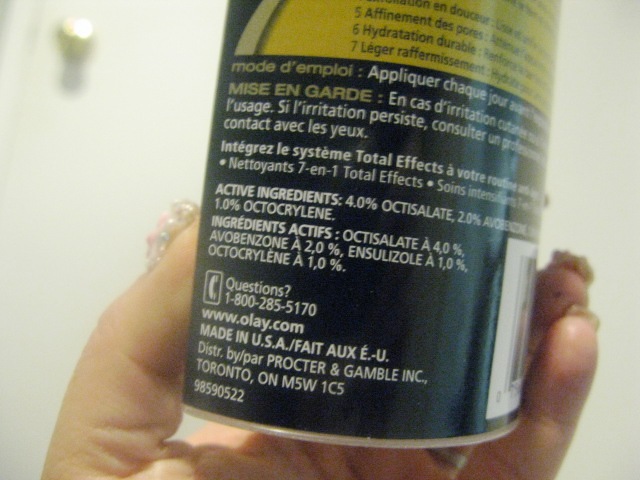The image features a close-up photograph of a person's hand holding a can. The can's top half is yellow with black text in French, and the bottom half is black with white French text. Keywords visible include "mode d'emploi" (apply every day) and "mise en garde" (in case of irritation). The ingredients listed are 4% octisalate and 2% of another ingredient. Part of the can's barcode and a contact number for questions, "1-800-285-5170," are also visible. The can is manufactured by Procter & Gamble. The background is white and somewhat blurry, with a small, shiny gold door handle visible in the top left corner. The person's hand is partially visible, with focus on their thumb, palm, and squared-off fingernails on two little fingers.